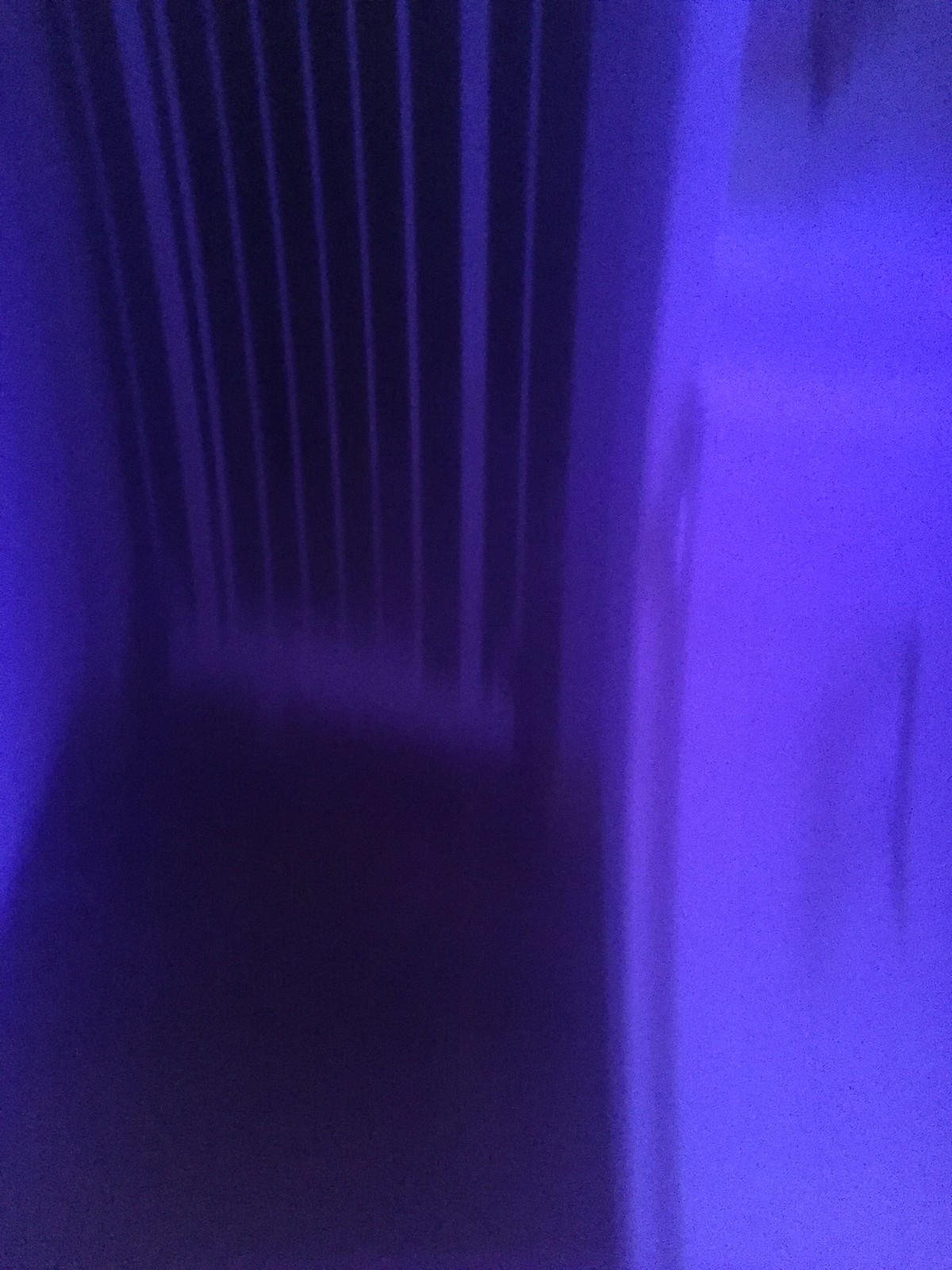This is a rectangular image featuring a tall white railed gate attached to the walls within a small entryway framed in white, situated in the top-left quarter of the image. The gate, with its center-opening mechanism, consists of almost seven or eight vertical bars, rendering the space between them pitch black, suggesting it could be nighttime or taken in a dark environment. The surrounding scene has a distinct purple or blue tint, akin to shades of lilac or dark purple. To the right side of the image, there is a white cabinet discernible by its hinges on the left and long handles, while the ground visible in the scene is dark gray. The overall perspective of the image appears slightly angled as if captured from a side view, peering across a ridge or possibly a light switch on a wall.